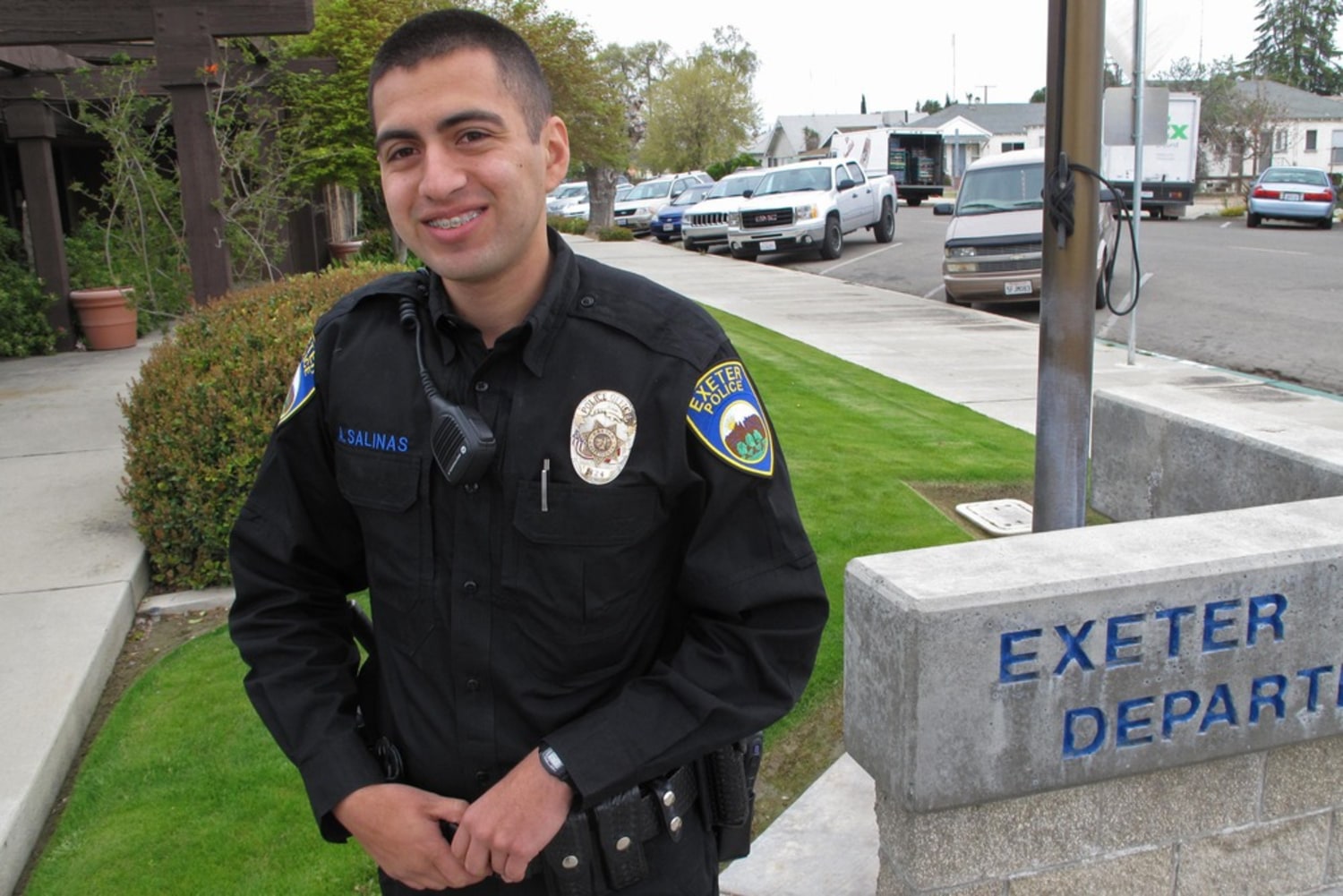In this color photograph, a young police officer, likely in his mid-20s, poses confidently in front of the Exeter Police Department. Standing on the front lawn, he is captured from head to waist in a landscape-oriented shot. The officer, identified by the name "Salinas" embroidered on his right shirt lapel in blue, sports a short, military-style black haircut and braces on his teeth. He is dressed in a black, long-sleeve uniform adorned with a shield-shaped patch on his left sleeve bearing the words "Exeter Police" in gold letters. His duty belt, equipped with ammunition, a holster, a walkie-talkie, and a shoulder-mounted mouthpiece clipped near his mouth, completes his professional attire. With his hands tucked casually into his belt, Officer Salinas smiles warmly at the camera. To his right, a low concrete sign inscribed partially with "Exeter Department" is visible, along with several parked cars in the background. The photograph, rich in photographic representational realism, effectively captures a moment of pride and professionalism in the officer’s career.